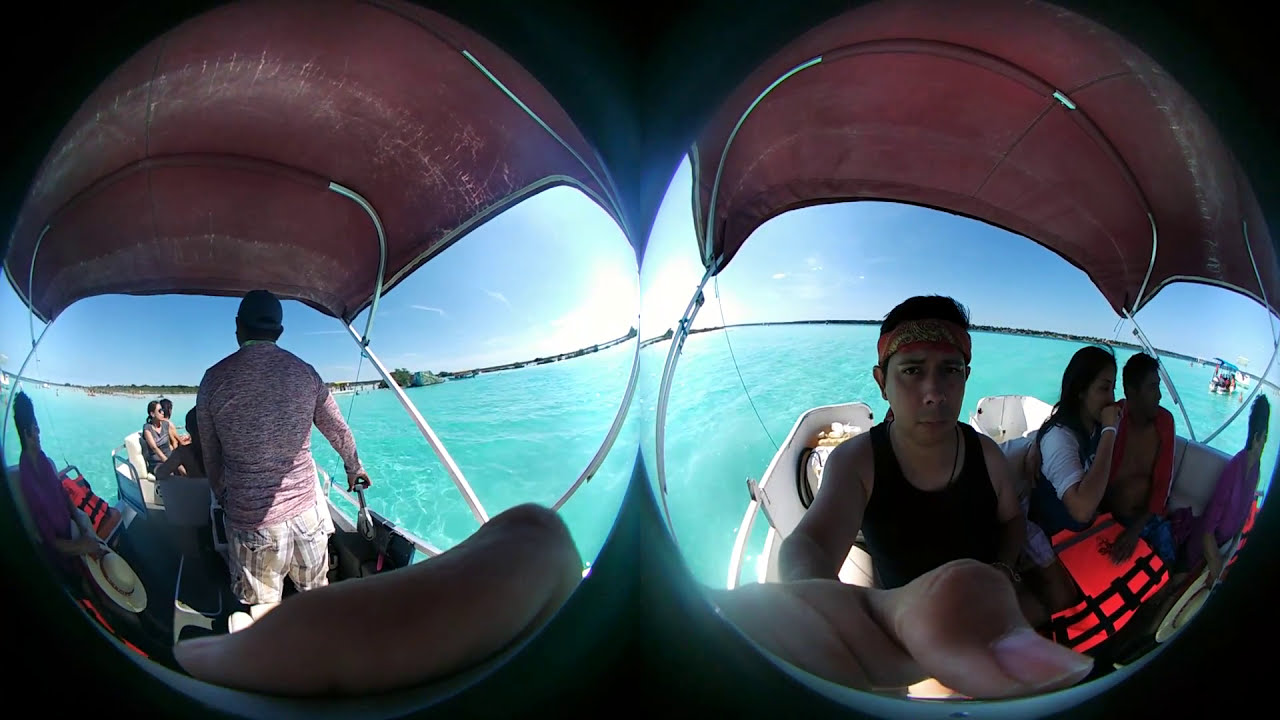This photograph presents a split image, with two rounded, contorted lens views side by side, providing a panoramic-like depiction of people on a boat. The backdrop comprises a tranquil turquoise blue sea with a faint horizon of trees and occasional man-made structures against a clear blue sky.

On the left section, centrally located, a middle-aged man in long sleeves and shorts, wearing a cap, is steering the boat. A woman in a purple shirt and straw-like sun hat is seated nearby, and you can glimpse additional passengers behind them. A small part of the image's bottom left shows the photographer's finger. Above, the maroon canopy of the boat is visible, offering shade.

The right section features a young man in a black muscle shirt and red headband, gazing neutrally at the camera. Three other people are in the frame, including a lady seated to his right, all against the backdrop of the steel-blue water. An orange life vest and the majestic open sea further define the scene, with a bit of land and vegetation peeking in the background.

This split image, with its dual spherical lenses, captures an array of details from the boat outing, blending individual expressions and shared experiences amidst serene aquatic surroundings.